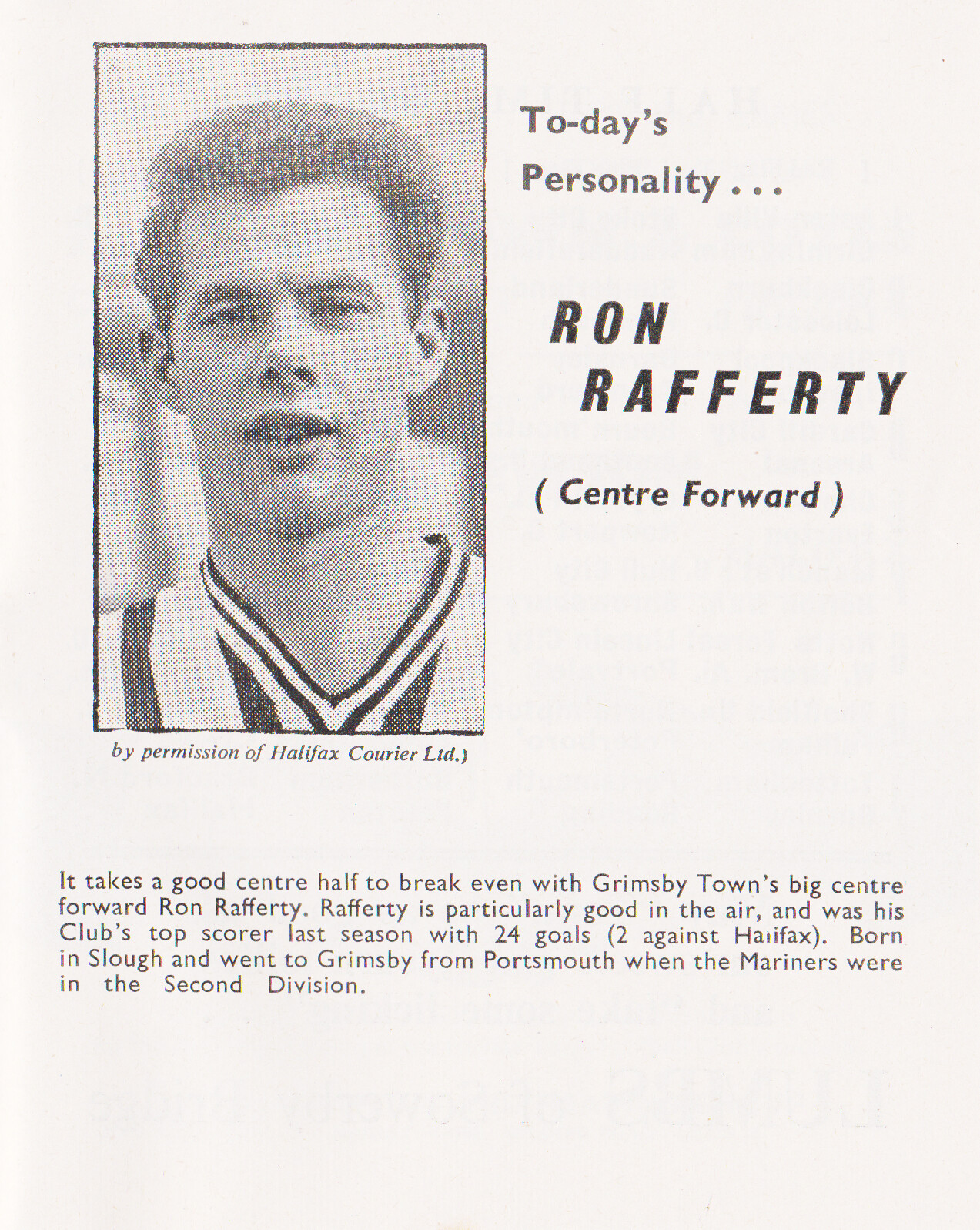The black and white image, likely from a newspaper or magazine article, features prominently in the center a photo of a male soccer player, Ron Rafferty. His mouth is slightly open, and he is dressed in a soccer t-shirt. To the right of the photo, bold text reads "Today's Personality… Ron Rafferty," with "center forward" in parentheses. Below the photo, a caption mentions the image is "by permission of Halifax Courier LTD." The accompanying text at the bottom of the image highlights Rafferty's prowess: "It takes a good center half to break even with Grimsby Town's big center forward Ron Rafferty." The text further details that Rafferty is particularly good in the air and was his club's top scorer last season with 24 goals, two of which were against Halifax. Born in Slough, Rafferty transferred to Grimsby from Portsmouth when the Mariners were in the second division. The flyer itself is white, with all the writing in black, set against what appears to be a gray background, resembling a magazine page.